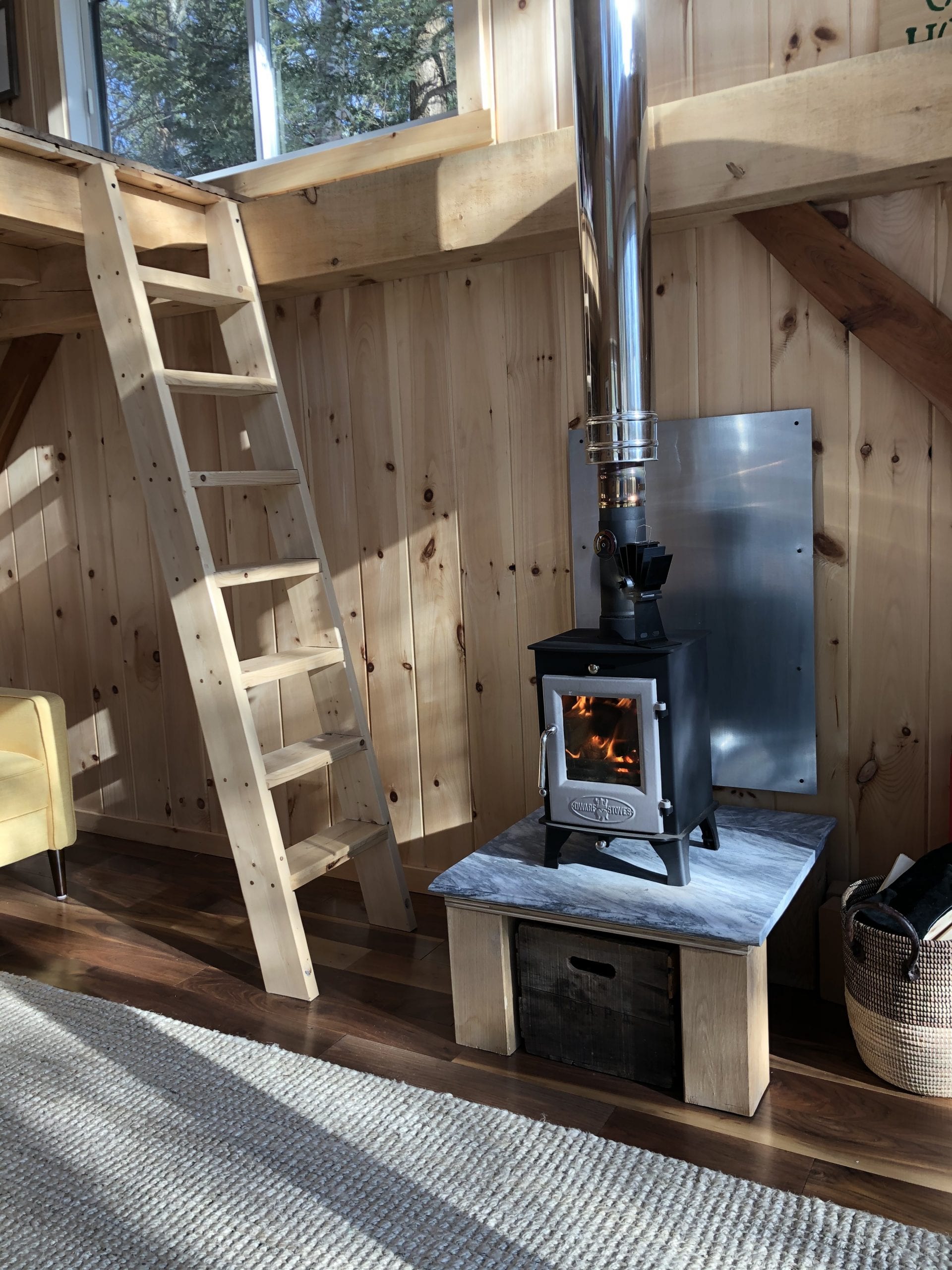The photograph captures the cozy interior of a compact wooden cabin. Central to the image is a small, black wood-burning stove with a front grey door featuring a large window, through which lit wood can be seen burning brightly. The stove rests on a raised platform with a distinctive white and black marbled surface. A large rectangular metal sheet mounted behind the stove acts as a heat reflector, safeguarding the surrounding light wood-paneled walls from damage. Extending from the top of the stove, a black pipe connects to a larger silver exhaust pipe that leads upwards towards the roof.

To the left of the stove, there's a wooden ladder leading to a second-story loft, adding to the vertical spaciousness of the compact area. Just visible on the far left side is the edge of a yellow chair, enhancing the room's inviting ambiance. The room is lit by natural light streaming in from a window on the right side of the image, illuminating the rugged yet charming features of the cabin. Below the stove, a grey carpet covers the floor, further contributing to the homey atmosphere. The unpainted wood walls retain their natural light brown hue, adding warmth and texture to the setting, which reflects a tight, enclosed, yet comfortable living space.